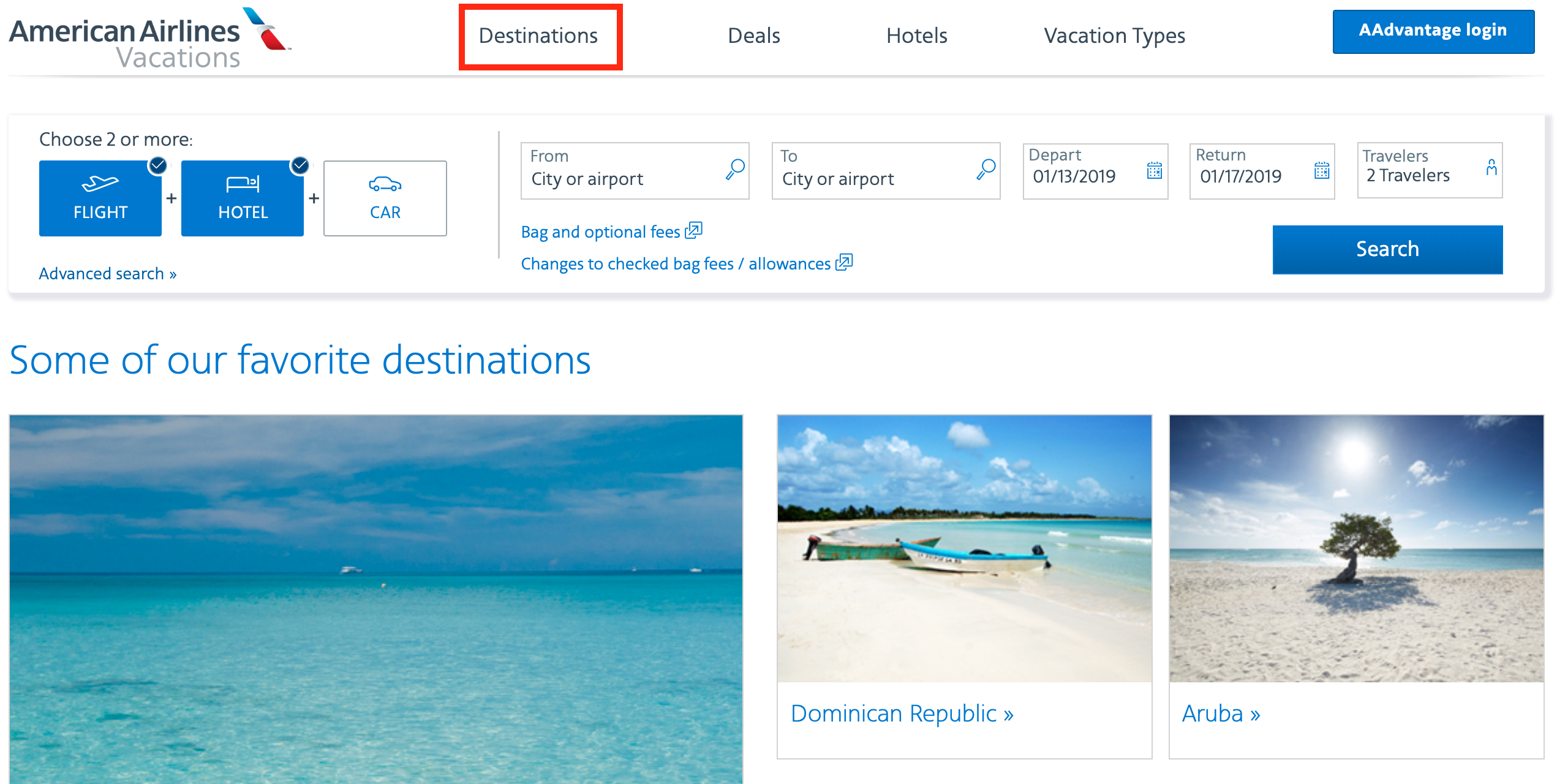This web page is from American Airlines Vacations. In the upper left-hand corner, the American Airlines logo is displayed in black, accompanied by an image of a red, white, and blue airplane. Beneath the logo, the word "Vacations" is prominently featured.

At the top of the page, navigation options include 'Destinations,' highlighted in a red box, along with other categories such as 'Deals,' 'Hotels,' 'Vacation Types,' and a login prompt labeled 'AAdvantage Login.' Below these, there is a section with the header 'Choose two or more.' This section features options for booking a flight, hotel, and car, with the flight and hotel options marked in blue and the car option in white. Users can enter their departure city or airport, select departure and return dates, and specify the number of travelers.

A blue search bar sits underneath this section, along with links to information about 'Bag and Optional Fees' and 'Advanced Search' options. Below this, there's a highlighted section titled 'Some of Our Favorite Destinations.' This section displays picturesque images: one featuring a beautiful turquoise sea under a partly cloudy blue sky, another showing a serene Dominican Republic beach scene with two boats, and a third image of an Aruba beach featuring a solitary tree.